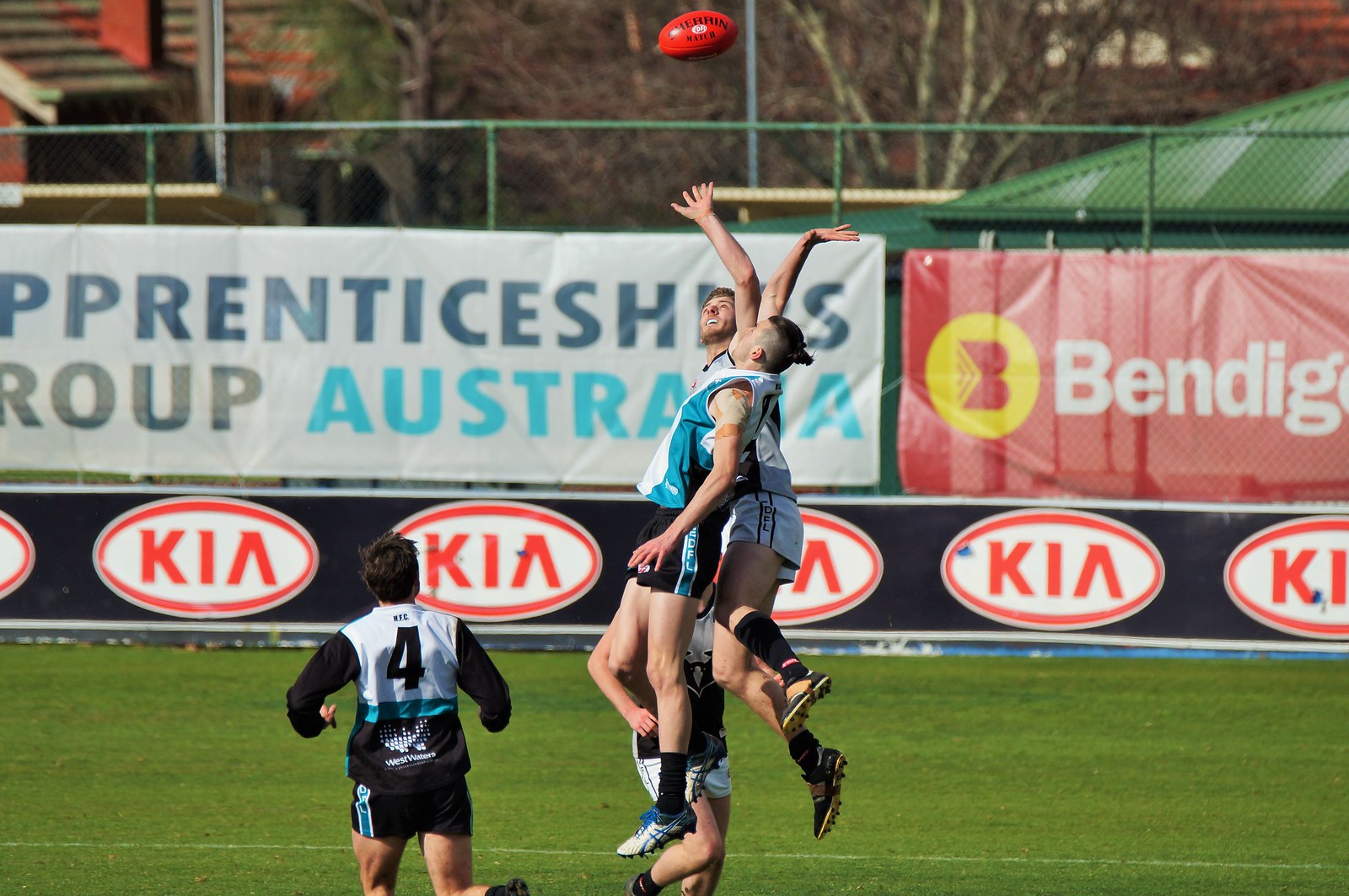The image depicts an intense rugby match with four players captured mid-action on a lush green field. Two players are seen leaping into the air, battling to gain possession of a red ball suspended above them—one attempting to catch it while the other tries to intercept. Both wear jerseys and shorts, with respective team colors of black, turquoise, and white, along with high socks and cleats. Below them, two other players are actively engaged in the play; one dashes towards the jumping duo while the fourth trails behind. The backdrop features a series of advertising banners affixed to a fence, notably including a white banner with blue and grey lettering promoting "Apprenticeships Group Australia," and a Kia advertisement with a black border displaying white and red lettering. Another vibrant red banner with yellow and white text is partially visible. The scene is set against a sunny sky, illuminating the competitive spirit of the game.